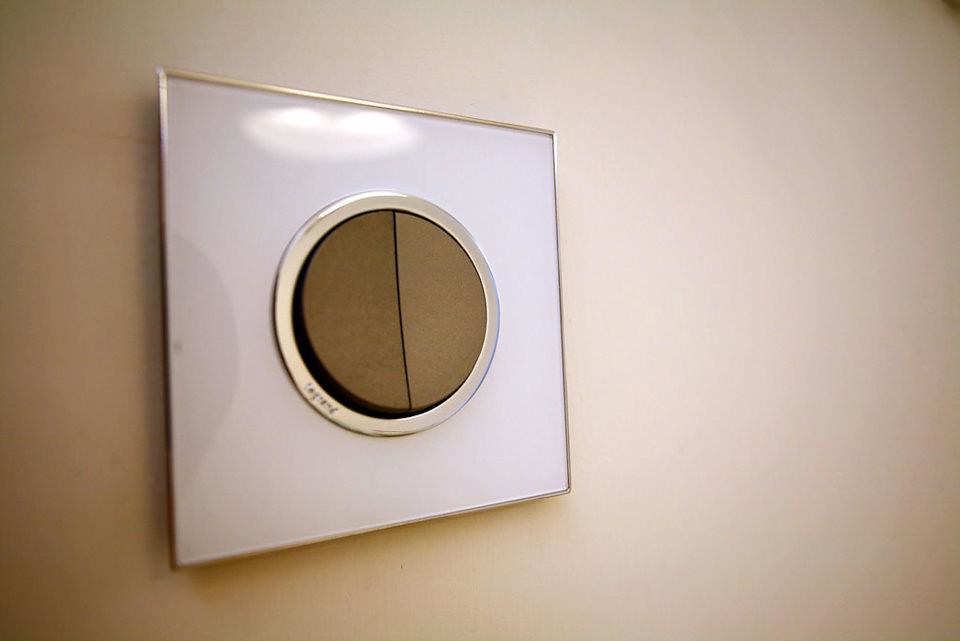The image showcases a photograph mounted on a white or beige wall, framed by a very thin, square, silver metal frame. The photograph’s background is stark white, and the glass surface reflects the surrounding light, creating a soft glare. Central to the photograph is a circle bordered by a shiny metallic ring, which casts a subtle shadow. Inside the circle, the space is divided into two distinct brown shades: a darker brown on the left and a lighter brown on the right. These two contrasting sections bear a resemblance to a makeup compact, possibly featuring eyeshadow or blush in two different shades. The rest of the photograph is devoid of additional elements, offering an empty and minimalist aesthetic.